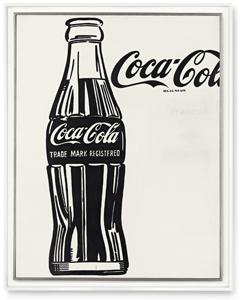The image is a rectangular photograph designed to sell a product, featuring a floating frame against a solid white background. This stylistic choice gives the appearance that the frame is hanging in an empty void, creating a stark and minimalist aesthetic typical of online listings for shops, catalogs, or websites. The frame contains a poorly fitted poster that is cut off on the right side, which detracts from its overall presentation.

The poster itself is a vintage Coca-Cola advertisement rendered in black and white. It depicts an old-fashioned Coca-Cola bottle, filled with soda up to the middle, and lacking a bottle cap. The iconic Coca-Cola logo is prominently featured in white cursive letters across the bottle. Below the main logo, the phrase "trademark registered" is written in smaller text. Adjacent to the bottle, partially cut off by the edge of the frame, the word "Coca-Co" is visible, with the remainder of "Cola" truncated. This area also includes some unreadable small text. The entire composition is bordered by a dark gray box, emphasizing the plain and unrefined nature of the image.